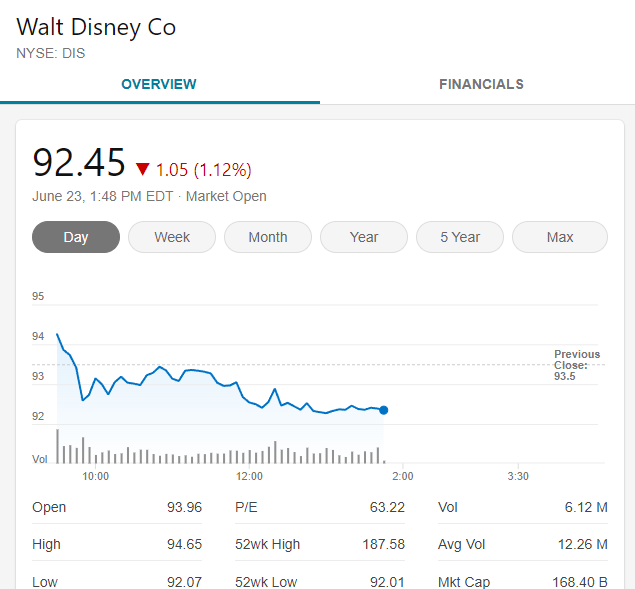Screenshot of Walt Disney Company Stock Overview:

This screenshot depicts the stock overview for the Walt Disney Company, listed on the New York Stock Exchange under the ticker symbol DIS. The information is predominantly displayed at the top in black text, starting with "Walt Disney CEO" followed by "NYSE: DIS" below it. 

The interface includes two clickable sections: "Overview" (currently selected and highlighted in blue with an underline) and "Financials." The overview section presents a snapshot of the stock's current performance.

Key details include:
- Stock price: $92.45
- Red downward-pointing triangle indicating a decrease: -1.05
- Percentage decrease: -1.12%
- Timestamp: June 23rd at 1:48 PM EDT (market open)

Below this, users can see options to view the stock performance across different timeframes, including "Day," "Week," "Month," "Year," "Five Year," and "Max." The "Day" option is currently selected.

The chart provides a visual graph of the stock's performance for the day. The vertical axis on the left is labeled with price markers: 95, 94, 93, 92. Additionally, the bottom left corner is labeled "Volume." The graph tracks the stock's movement from 10:00 AM to 3:30 PM, with time markers at 10 AM, 12 PM, 2 PM, and 3:30 PM.

Additional statistics listed at the bottom include:
- Open
- High
- Low
- Volume
- Average Volume
- Market Cap

These numbers provide a comprehensive overview of the stock's performance and market activity for the given day.